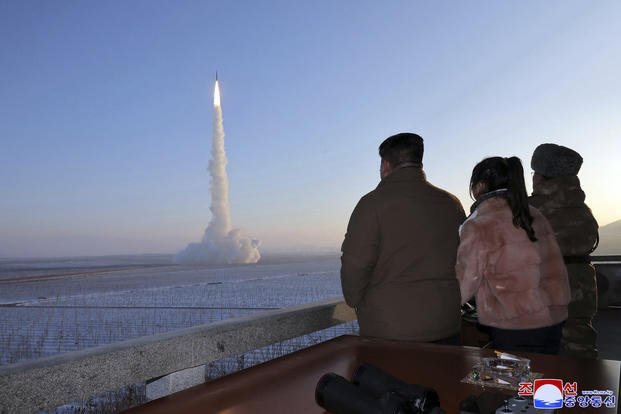The image captures a dramatic scene of a rocket launch viewed by three distinct figures. On the right side of the photograph, standing on a podium high above a vast, snow-covered field, are three people believed to be significant, possibly political figures from North Korea. The man closest to the viewer, who appears to be Kim Jong-un, the leader of North Korea, is heavyset with short black hair, wearing a brown coat. Beside him, a woman with long black hair dons a fuzzy pink fur coat, and next to her, another individual is clad in olive-green camo winter clothing and a round gray fuzzy hat. The table in front of them holds a pair of black binoculars, likely used to observe the launch more closely. Stretching out from the horizon is the expansive snowy field leading to the spectacular event of a rocket lifting off into the sky. A massive cloud forms at the base of the launch, trailing the rocket with a stream of white smoke as a bright flame propels it upward. The remote location, free from any structures and marked by sparse grass shoots and a watery area in the foreground, emphasizes the isolation and grandeur of this momentous occasion. Hangul characters in red, white, and blue at the bottom right hint at the Korean context of the image.